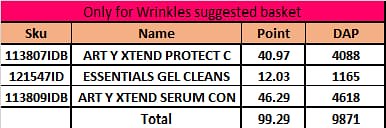The image depicts an Excel spreadsheet meticulously organized into four columns and six rows, focused on body care products. The first row is highlighted with a magenta background and bears the title "Only for wrinkles suggested basket," enclosed in a red outline. The second row serves as the header for the following columns, with cell backgrounds in a light orange hue. The columns are labeled: SKU, Name, Point, and DAP (all in uppercase). The subsequent rows list specific product details:

1. **SKU 1138071DB** – *Art Y Extend Protect C*: 40.97 points, 4088 DAP.
2. **SKU 121547ID** – *Essentials Gel Cleans*: 12.03 points, 1165 DAP.
3. **SKU 113809IDB** – *Art Y Extend Serum CON*: 46.29 points, 4618 DAP.

The table concludes with a row indicating the total points and DAPs, summing up to 99.29 and 98.71, respectively.